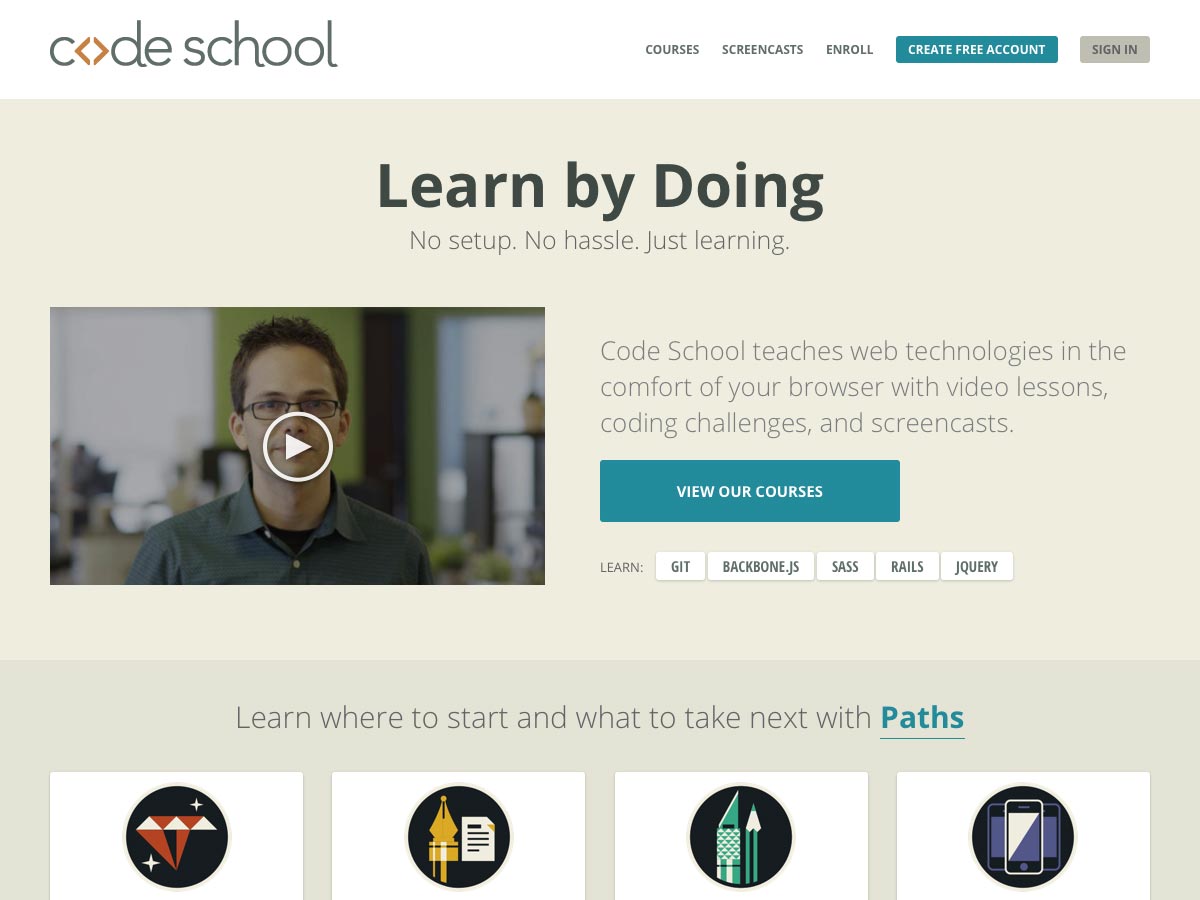This image depicts a website for "Code School." In the upper left corner, the site's logo displays the words "Code School," with the "O" styled as an orange diamond, while the other letters are black. On the right side of the header, green text invites users to "Create Free Account," next to options to "Sign In," "Enroll," "Screencasts," and "Courses."

Central to the layout is a tan box that prominently declares "Learn by doing" in bold black letters. Below this, the phrases "No setup, no hassle, just learning" are displayed. Beside this text is a photograph of a white man with brown hair wearing glasses and a gray button-down shirt. There is a circular play button near his mouth, represented by a white arrow within a circle, indicating a clickable video.

Adjacent to the man's image, a text block reads, "Code School teaches web technologies in the comfort of your browser with video lessons, coding challenges, and screencasts. View our courses." Below this, a green bar lists technologies such as "GIT, Backbone, Sass, Rails, and jQuery."

Under this section, a darker gray box features a green text stating, "Learn where to start and what to take next with paths." The box includes four black circles, each containing distinct icons: a red and white diamond, a gold pointy shape resembling a rocket ship, a green set of pencils, and a purple-bordered phone.

The design and information elements collectively convey that this website is dedicated to teaching web technologies through interactive and comprehensive learning paths.